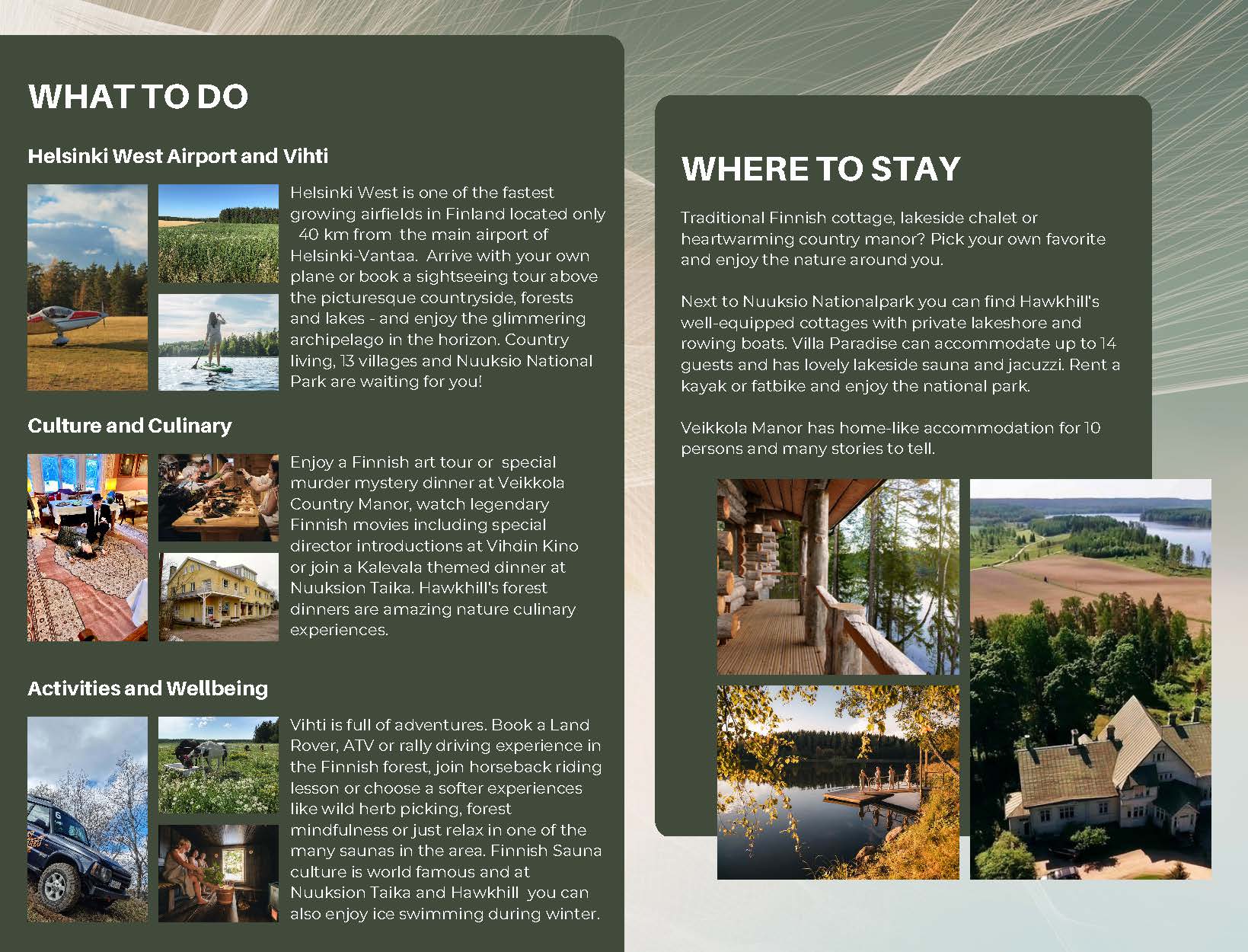**Discover Helsinki West: A Unique Finnish Getaway**

Immerse yourself in the charm of Helsinki West, one of Finland's fastest-growing regions just 40 kilometers from Helsinki-Vantaa Airport. Nestled amidst picturesque countryside, lush forests, and serene lakes, this destination offers a perfect blend of adventure, culture, and relaxation.

**Travel & Arrivals:**
Experience the thrill of arriving at Helsinki West, either by your private plane or through a scenic sightseeing tour in a small aircraft. The heliport caters to aviation enthusiasts and those eager to explore Finland's natural beauty from above, offering breathtaking aerial views of the countryside.

**Activities & Wellness:**
- **Adventure:** Engage in exhilarating activities like Land Rover ATV rides or rally driving through dense forests. For a softer adventure, enjoy horseback riding sessions amidst the tranquil Finnish landscape.
- **Relaxation:** Embrace nature with wild herb picking or forest mindfulness sessions. Unwind in one of the many traditional Finnish saunas, a quintessential part of the local experience.

**Culinary & Cultural Delights:**
- **Food Experiences:** Savor unique culinary experiences such as a forest dinner at Aakhil or a Kalativa-themed feast at Nuukasoo Takawa. Indulge in a special murder mystery dinner at Biokal Country Manor or relish the ambiance of local restaurants where joyous high-fives set the tone.
- **Art & Film:** Take a Finnish art tour or watch legendary Finnish movies, immersing yourself in the country's rich cultural tapestry.

**Country Living & Nature:**
- **Villages & Parks:** Discover the essence of Finnish country living across 13 charming villages and the expansive New Sikko National Park.
- **Scenic Spots:** Explore the verdant fields and capture moments paddleboarding in scenic lakes, offering an idyllic respite from urban life.

**Where to Stay:**
- **Accommodation Options:** Choose from traditional Finnish cottages, lakeside chalets, or grand country manors. Each offers a unique stay – cozy log cabins on serene lakeshores with private docks, or luxurious manors with sweeping aerial views, ensuring a perfect retreat for every traveler.

Helsinki West promises a blend of thrilling adventures, serene landscapes, rich culture, and unparalleled relaxation, making it a must-visit destination for every traveler.